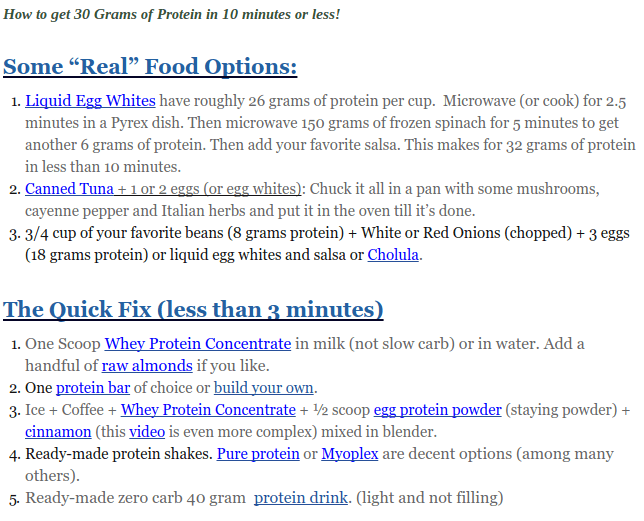In the image, we observe a recipe webpage from what appears to be a fitness-focused site with a clean, white background. At the top of the image, the heading reads "How to Get 30 Grams of Protein in 10 Minutes or Less."

This is followed by two sections. The first section, titled "Real Food Options," lists three suggestions:

1. Liquid Egg Whites - Accompanied by detailed information about the protein content.
2. Canned Tuna plus 1 or 2 Eggs/Egg Whites - Offers guidance on combining tuna with eggs for a protein-rich meal.
3. 3/4 Cup of Your Favorite Beans - Presented as another viable option.

The second section, labeled "Quick Fix (Less than 3 Minutes)," provides five fast solutions:

1. One Scoop of Whey Protein Concentrate.
2. One Protein Bar.
3. Iced Coffee plus Whey Protein Concentrate plus One Scoop of Egg Protein Powder.
4. Ready-Made Protein Shakes.
5. Ready-Made Zero Carb Protein Drink.

Each section provides practical and time-efficient approaches to reaching a daily protein goal, catering to both real food enthusiasts and those in need of quicker solutions.